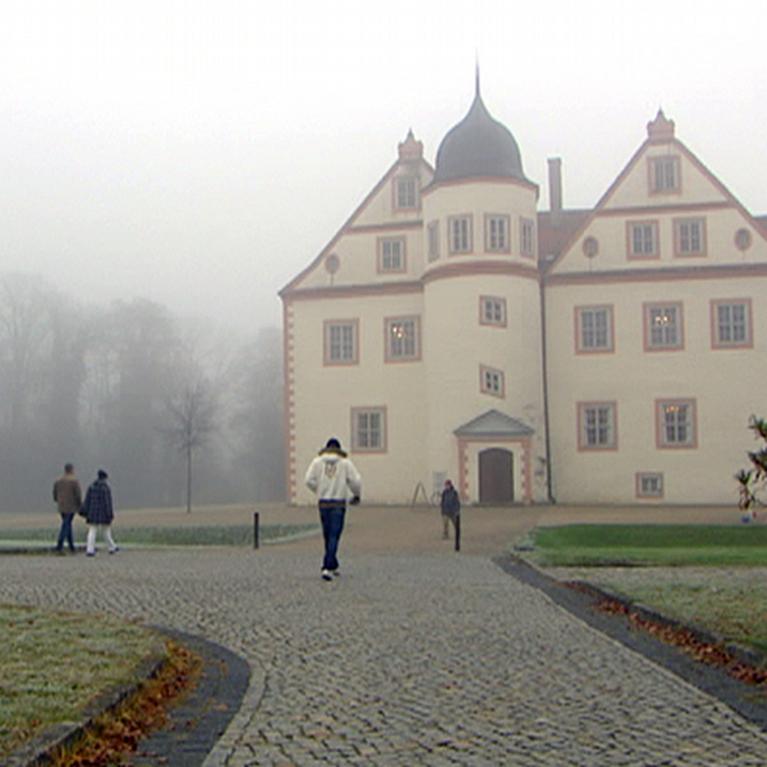This photograph captures a misty, overcast day outside a large, cream-colored building that exhibits European architectural style. The building features sloping rooftops and a distinct dark-grey dome with a pointy tip, which sits atop a temple-front entrance. The facade is dotted with many windows framed in brown wood, set against beige walls that appear to be made of stucco or plaster. The building also has red highlights and a pair of pitched roofs on either side of the central dome. 

People dressed in warm winter clothes, including coats and jeans, walk along a grey, paved walkway made of brick pavers. Some are approaching the building, while others are leaving. The entrance door is a dark brown double wooden door. A green patch of grass flanks both sides of the walkway, complemented by trees and plants. 

The mist or fog is more pronounced on the left side of the image, partially obscuring the trees, which have brown and red leaves scattered around the grey concrete curb. The atmosphere is further characterized by a hazy, white or grey sky, giving the overall scene a cold, foggy ambiance.